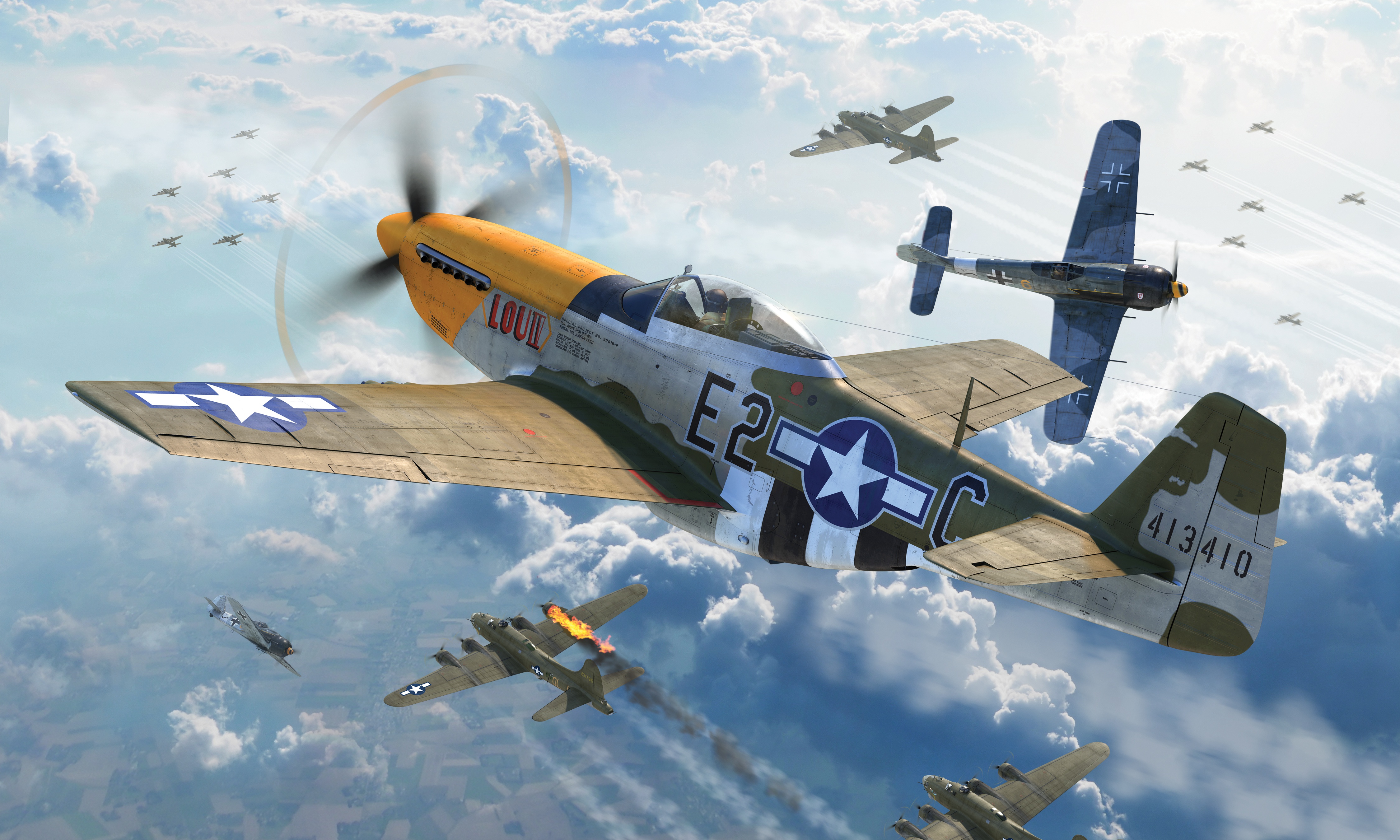This image appears to be a screenshot from a video game or a CGI render, depicting a formation of World War II-era military airplanes soaring high in a vibrant sky filled with various shades of blue, white, and gray clouds. Numerous aircraft, some appearing closer than others, fill the scene, characterized by their green and gray color schemes, along with distinctive markings including blue circles with white stars on the wings and fuselages. The leading plane features a yellow nose and a visible cockpit occupied by a pilot, with red text and additional silver detailing. Identifying numbers such as "E2" and "413, 410" are visible on the side and tail of the aircraft. Notably, one of the planes in the background appears to be on fire, with striking yellow, orange, and red flames. Below, the ground is just visible in the bottom left corner, showcasing patches of brown and green land. Overall, the composition captures a moment of dynamic aerial action set against a richly textured sky.